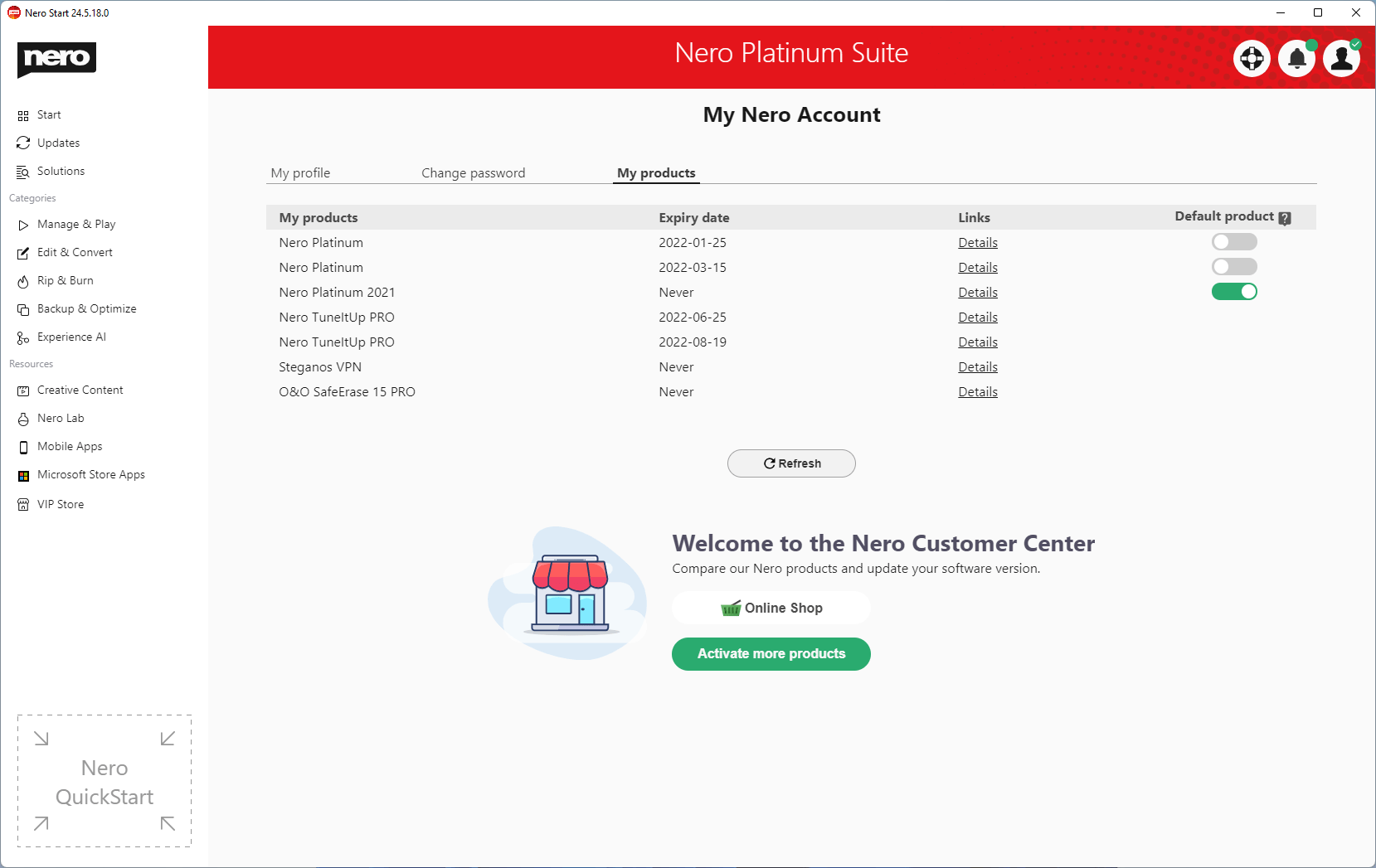The image displays a webpage showcasing the Nero Platinum Suite. At the top, a prominent red bar bears the text "Nero Platinum Suite," while a smaller black bar on the left displays the word "Nero." Below the red bar, a sidebar menu lists various options: Start, Updates, Solutions, Manage and Play, Edit and Convert, Rip and Burn, Backup and Optimize, and Experience AI. Further down, additional resources are available, including Creative Content, Nero Lab, Mobile Apps, Microsoft Store Apps, and the VIP Store.

In the central part of the page, a section titled "My Nero Account" is visible. It offers sub-options like My Profile, Change Password, and My Products. Under "My Products," the user can view a detailed list of products included in the Nero Platinum Suite, such as Nero Platinum, Nero Platinum 21, and Nero TuneItUp Pro, along with their respective expiry dates. Each product entry includes a "Details" link for more information and a "Default Product" toggle button to set a specific product as default. 

On the far right, there are options to refresh the page, along with a welcome message to the Nero Customer Center. This section also provides tools to compare different Nero products, update the software version, visit the online shop, and activate more products. In the top right-hand corner, icons for the user's profile, notifications, and settings are clearly visible.